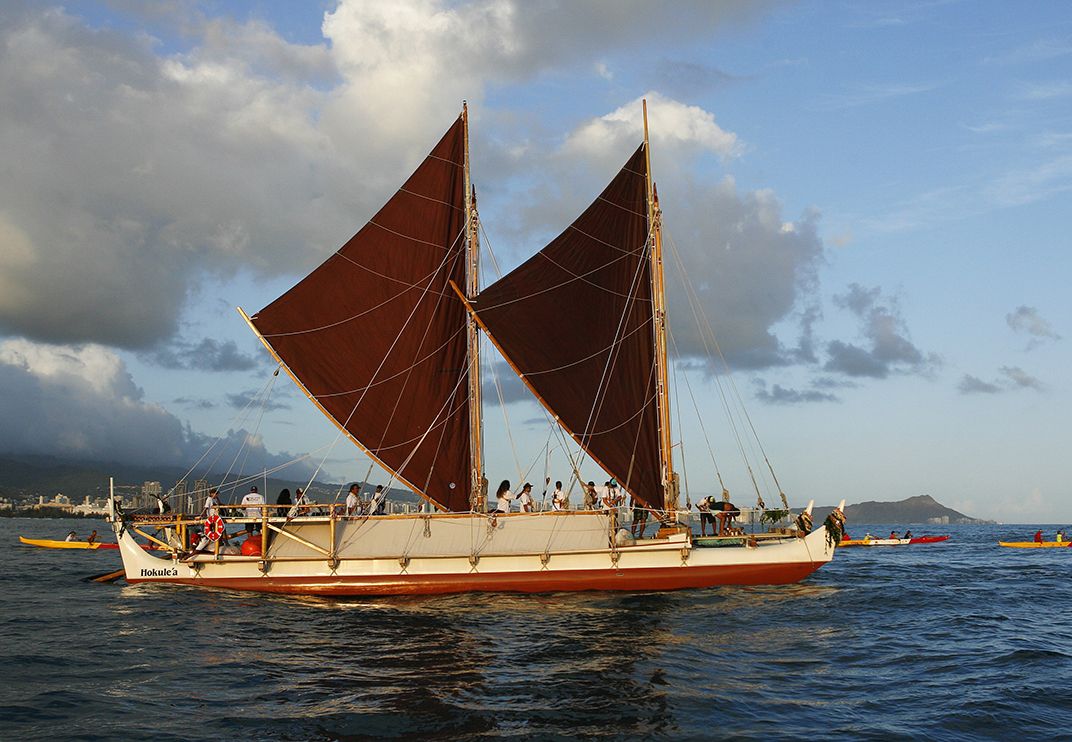In this daytime image taken on a vast body of water, a large sailboat named "Hōkūlae‘a" with distinctive dark burgundy sails and a light tan wooden mast is prominently featured. The boat, which has a white hull with red at the bottom, is bustling with approximately 40 people who appear to be enjoying a party or tour. They are standing and looking out to the sides, some holding cocktails. Surrounding the sailboat are several smaller tropical-style canoes, each seating two people, and painted in vibrant yellow, red, and white colors. The sky above is mostly blue, dotted with patches of gray clouds, suggesting a partly overcast day. In the distance, a coastline with mountains and structures, including hotel buildings, can be seen, enhancing the tropical atmosphere of the scene.